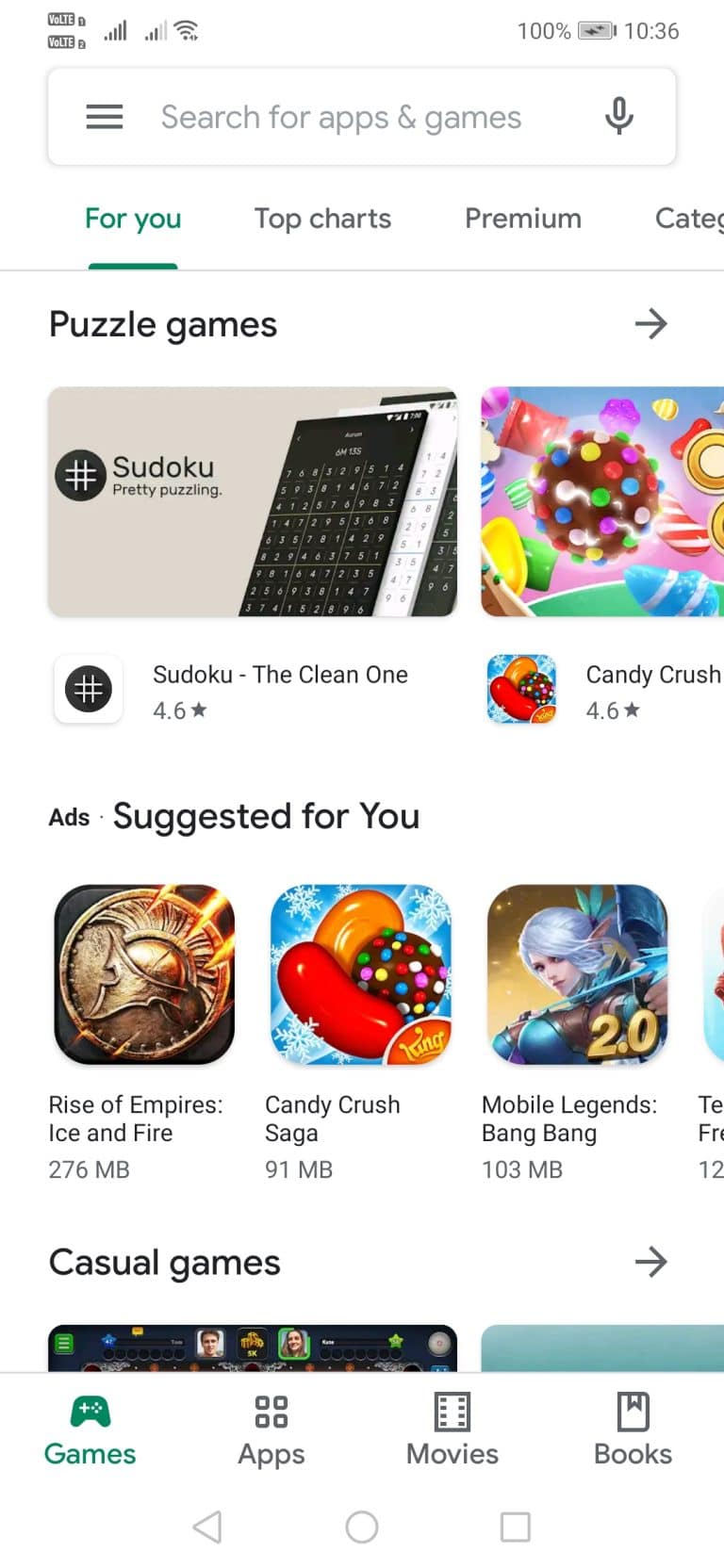A detailed, cleaned-up caption for the described image could be:

This is a color screenshot of a mobile device screen displaying a page from an app store. In the top left corner, there are two battery icons labeled "VoLTE," indicating signal strength; the first shows full bars, and the second has three bars. Adjacent to these, a full Wi-Fi signal is displayed alongside a battery icon indicating 100% charge at 10:36 AM.

The search bar at the top of the screen reads "Search for apps & games." Below it, menu options are listed: "4U," "Top charts," "Premium," and partially cut-off "Categories," with "4U" highlighted in green and underlined. 

The next section features the label "Puzzle games" in black text, accompanied by a right-facing arrow on the right side. Underneath this, a color image depicts a grey background featuring the text "Sudoku - Pretty Puzzling." The image includes two Sudoku puzzles, one black and white, leaning against each other. Below, the app is described with the text "Sudoku - The Clean One" rated at 4.6 stars. 

Next to it is the "Candy Crush" app, featuring a colorful box with purple and blue highlights, various candies, and the iconic Candy Crush sphere with multi-colored dots. It is also rated at 4.6 stars and includes the app icon.

Further below, an "Ad - Suggested for you" section lists additional apps:
- "Rise of Empress: Ice and Fire" (276 MB)
- "Candy Crush Saga" (91 MB)
- "Mobile Legends: Bang Bang" (103 MB)

Each app is accompanied by its icon. The final section shows a category called "Casual games" with a right-facing arrow, followed by additional categories: "Games," "Apps," "Movies," and "Books."